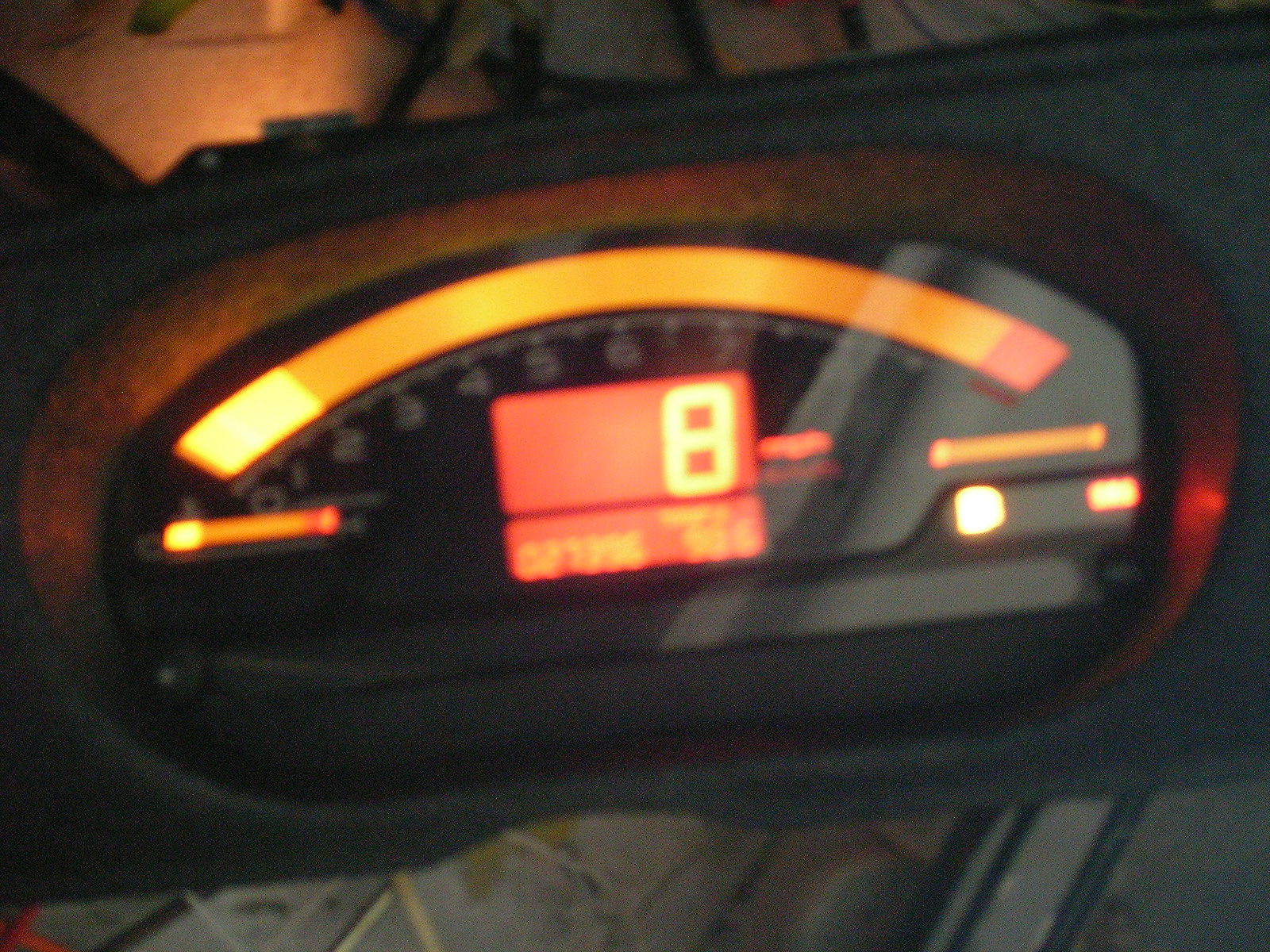This image is a close-up of a rounded electric meter encased in a black housing with a black front panel. Central to the image is a small rectangular digital display showing the number "8" in red. Below this primary display is a smaller, less discernible digital display due to the photo's blurriness. To the left of the central display, an orange line is illuminated, with the brightest segment of this orange line at the far left. At the top of the meter is a thick, semicircular line accompanied by curved numbers ranging from 1 to 7, but a glare obscures the numbers on the right side. There are two illuminated lights on the bottom right corner of the meter, one positioned slightly left and the other to the right. In the top left corner of the image, an orange light glows in the background. Lower in the photo, pieces of wire can be seen on the left, and a piece of metal, seemingly attached to concrete, appears in the bottom right.